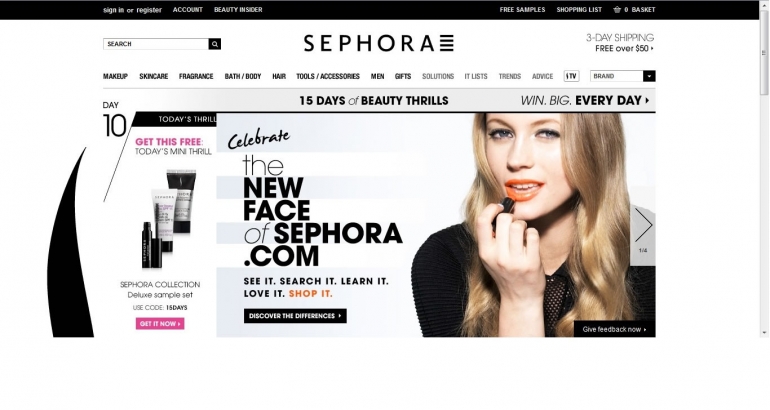Screenshot of a Sephora Web Page: 

The page features a clean white background with a sleek black banner stretching across the very top. This banner contains white text listing options: "Sign In or Register," "Account," "Beauty Insider," a space, followed by "Free Samples," "Shopping List," and a basket icon indicating zero items labeled "Basket."

Centered below this banner, the brand name "Sephora" is boldly displayed in black text, with four stacked lines beneath it. To the left of this brand name is a prominently placed search bar. On the right side of the brand name, there’s a message about "Three-day Shipping Free over $50," accompanied by a directional arrow.

The menu bar beneath this mentions, from left to right, categories like "Makeup," "Skincare," "Fragrance," "Bath/Body," "Hair," "Tools/Accessories," "Men," and "Gifts." In a gray section slightly lower, it lists "Solutions," "Trends," "Advice," "TV," followed by another search bar and a "Brand" dropdown menu.

Prominently displayed beneath this section is a promotion for "Day 10" of a 15-day beauty event, featuring "Today's Thrill": a free Sephora Collection Deluxe Complete Set using the code "15DAYS." This is highlighted on a hot pink rectangle with white text reading "Get it now." Next to it are two tubes and a mascara, with additional text promoting "15 Days of Beauty Thrills."

Below this is a celebratory message: "Celebrate the new face of Sephora.com. See it, search it, learn it, love it, shop it." Adjacent to this, a striking black rectangle with white text encourages users to "Discover the differences."

To the right, an image features a Caucasian woman with long blonde hair, blue eyes, and a black mesh-style shirt applying orange lipstick. She faces the camera directly, and beside her is a directional arrow pointing right. At the bottom right, there’s a black rectangle prompting users to "Give Feedback Now" in white text.